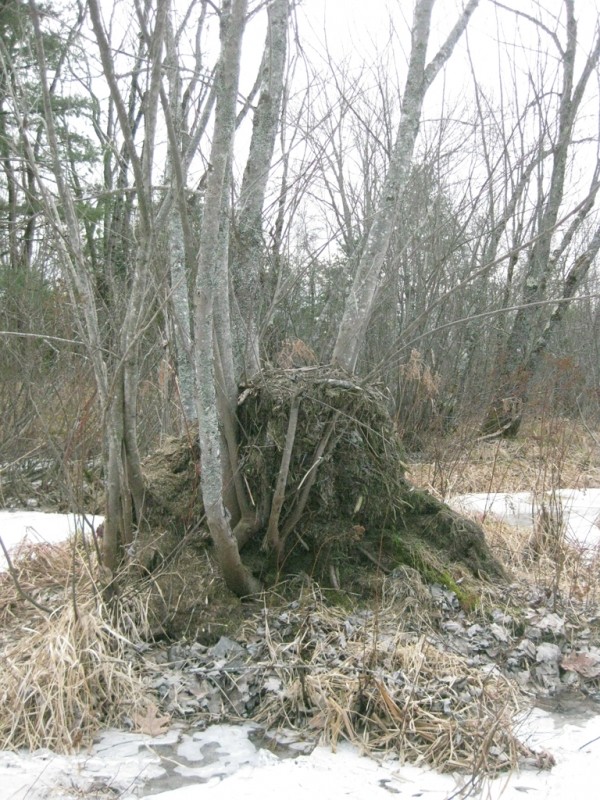The photograph captures an outdoor natural setting, focusing on a central tree surrounded by a mound of soil that has turned grayish due to algae growth. The soil heap, which seems to connect multiple tree trunks at their bases, gives the illusion of a single large tree. Extending from the mound is a network of gray stems reaching outwards and upwards. The ground around the mound is scattered with brown and gray dry leaves and shoots, amidst which lie dried grasses and rocks. A light layer of snow is evident on the ground and in the background, where more trees extend into the distance. The white sky is visible through gaps in the tree stems. Adding to the scene’s complexity, a barely visible river meanders through, enhancing the forest-like ambience filled with branches, sticks, and diverse plant life.